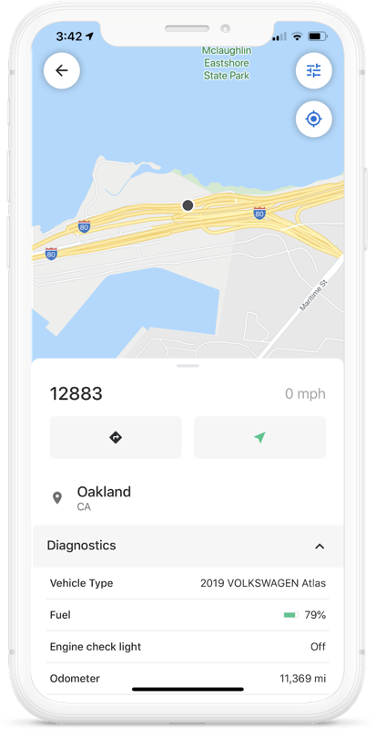A white modern phone with rounded edges, potentially an Apple device, is depicted in this image. The phone’s screen displays a map application. Toward the upper middle of the device, there is a small slit, likely for the earpiece, and to its right is a small circle that may house a front-facing camera. On the top left of the screen, "3:42" is displayed, likely the time. Next to it, there is a black send arrow, followed by a signal strength icon showing two out of four bars, a Wi-Fi signal icon at half strength, and a battery icon that is about three-quarters full.

Beneath these indicators, on the left, there is a white circle with a left-pointing arrow, presumably a back button. The main screen shows a map focused on McLaughlin East Shore State Park, though part of the text is cut off. There's a circular settings icon that resembles a target or location pinpoint. A black dot, possibly indicating a destination or current location, is positioned on a highway section within the map display. Various routes and bodies of water are visibly mapped.

Below the map, the number "12883" is displayed, followed by two rectangular buttons. The bottom of the screen shows a location marker icon, with the text "Oakland, CA" underneath it. Additional information at the bottom includes tabs or selectable options: "diagnostic" (highlighted), "vehicle type," "fuel," "engine check light," and "odometer."